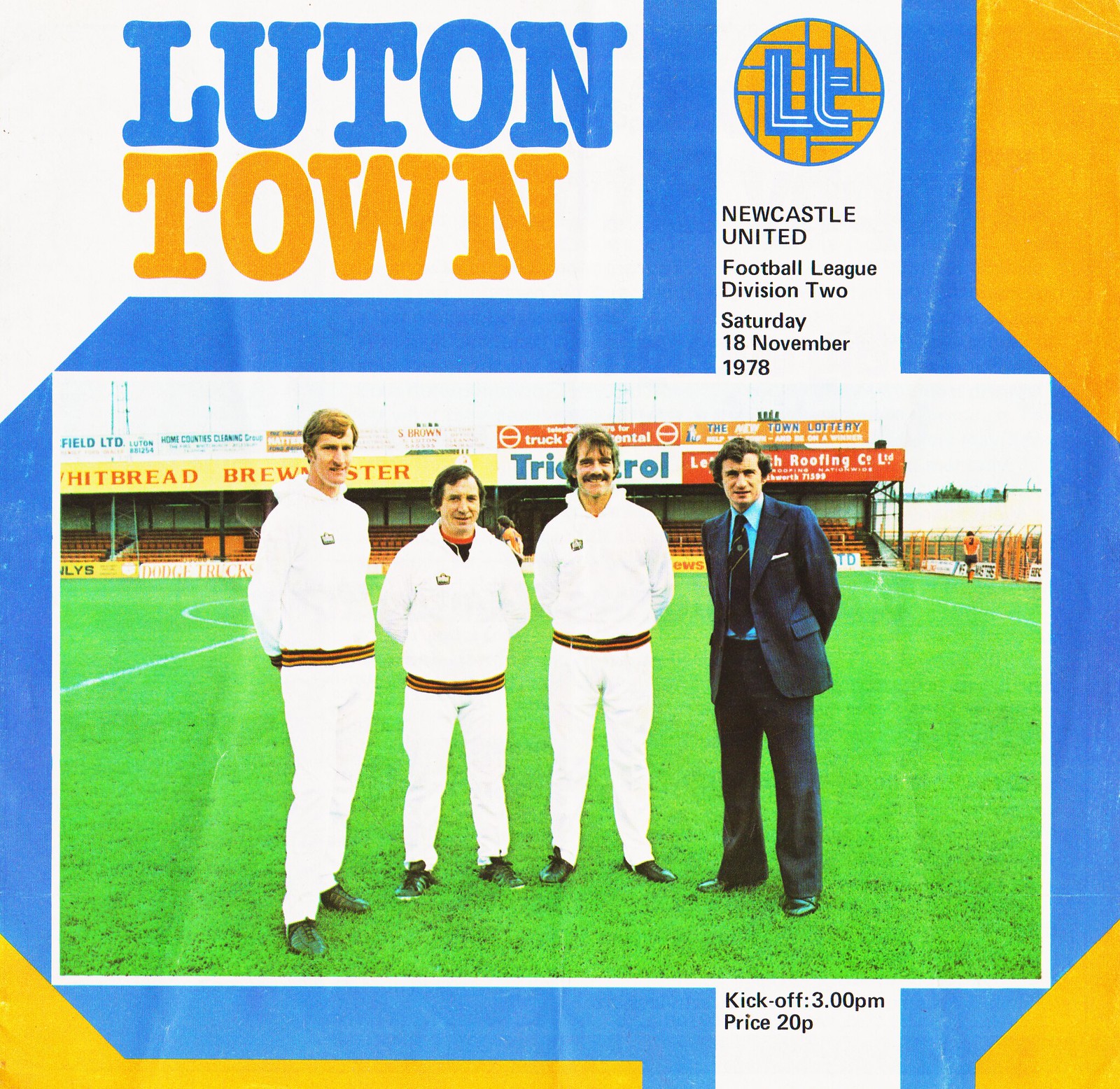This image depicts the front cover of an official match program for a European professional football club. Dominating the top left corner in large, capital blue letters, it reads "LUTON," with "Town" beneath it in capital yellow letters. Adjacent to this on the top right is the Luton Town logo, featuring blue letters within a sort of yellow circle. The text underneath announces the match against Newcastle United in the Football League Division 2, scheduled for Saturday, 18th November 1978.

Central to the image are four figures standing on a grass football field, looking directly at the camera. Three of the individuals are dressed in white tracksuits with orange and black waistbands, likely football players or coaches, while the man on the far right is clad in a navy blue business suit, complete with a light blue shirt and a matching tie. Surrounding them in the background are various advertising signs for companies such as Whitbread Brewsters and a roofing company.

The bottom of the cover is marked with the details "kickoff 3 p.m., price 20p," and the overall color scheme includes shades of white, blue, orange, black, light blue, yellow, red, and green, reinforcing the vintage aesthetic of this 1978 football program cover.